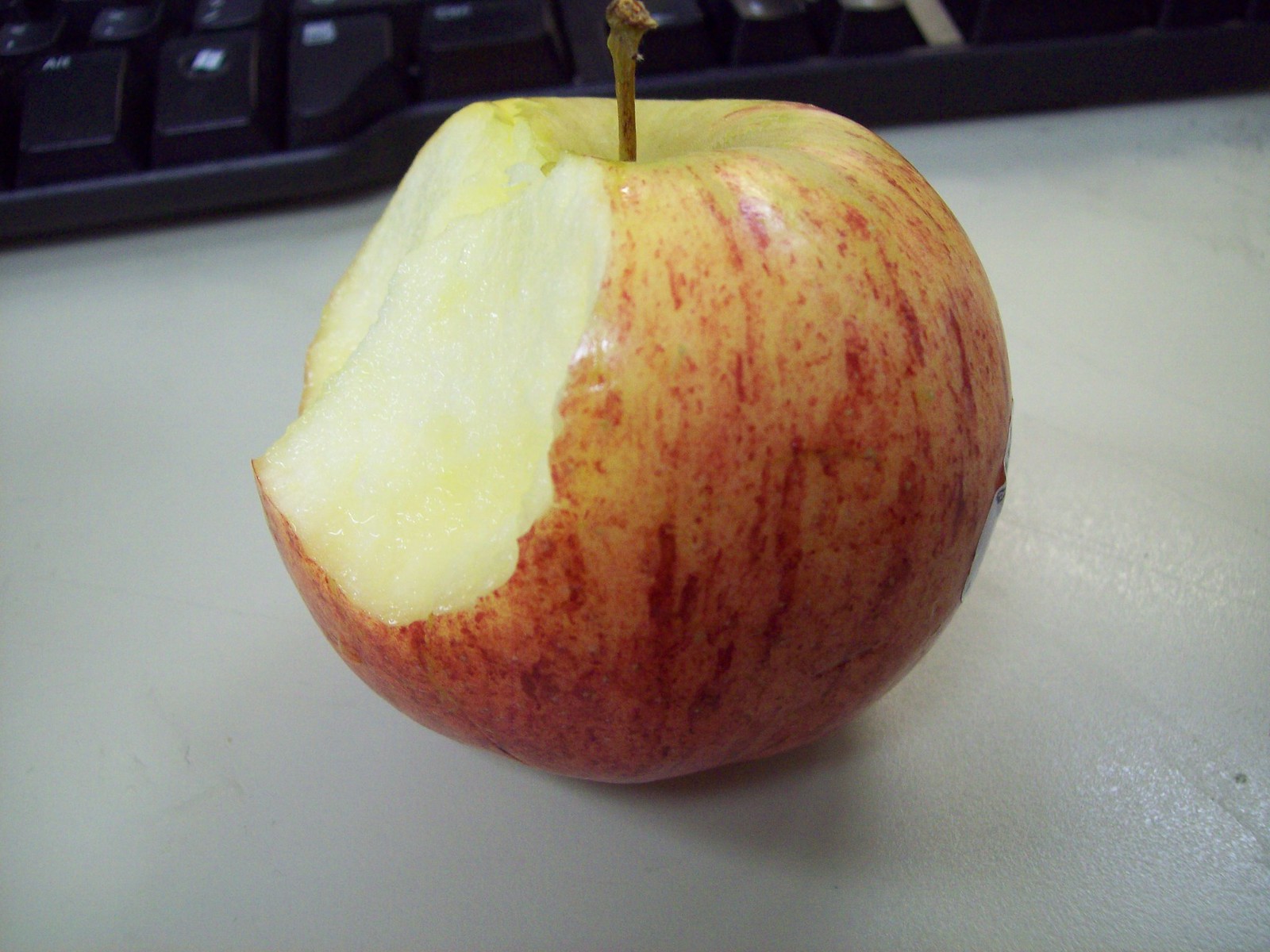This image features a red and green-speckled apple resting on a pristine, white marble surface. A bite has been taken out of the apple on its left side, revealing its white, juicy interior. The apple has a green stem protruding from the top. In the upper background, a portion of a black keyboard is visible, specifically showing the Alt and Windows keys. Shadows from the apple and the keyboard are cast onto the marble surface, adding depth to the composition. The apple appears to be only halfway ripe, with its speckled skin and crisp interior on display.